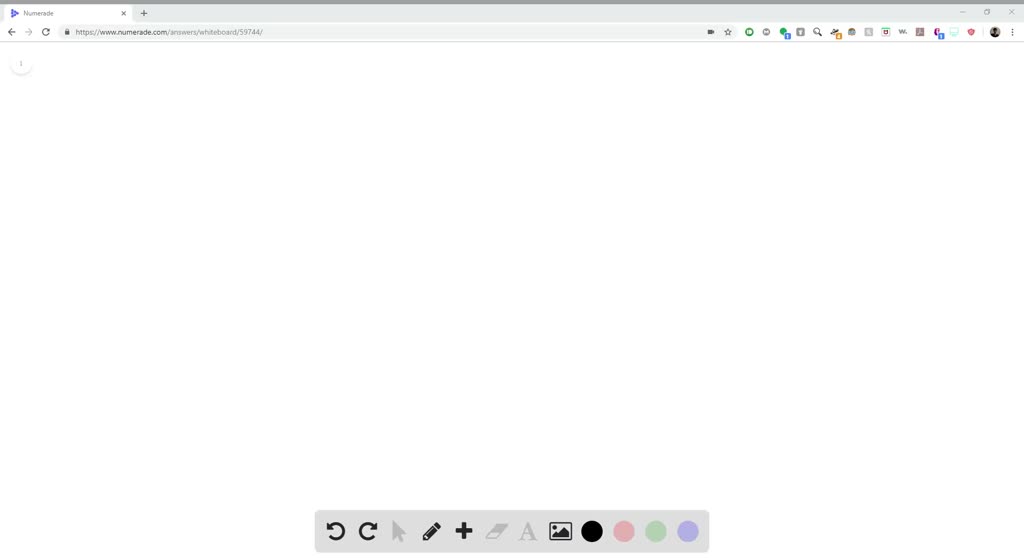This screenshot captures the top portion of a web browser, showcasing the address bar, tabs, and a set of icons. The featured tab is labeled "numerate," identifying it with a unique icon: a purple triangle composed of smaller circles. The address bar displays a padlock icon next to the secure URL "https://www.numerate.com." Adjacent to the address bar, on the right side, is a series of icons, concluding with the user's avatar on the far right. 

The webpage itself appears blank, with a white background and no visible content. Below the tab labeled "numerate," there's a gray number "1" encircled by a light ring, indicating an unseen notification or item count.

At the bottom center of the browser, a toolbar offers various customization options. This bar includes icons for editing and adding elements to the page: a pencil icon for drawing or annotating, a plus icon for adding new elements, an insert photo icon, and three colored circles (black, pink, green, and lilac) presumably for color selection. Some icons within the toolbar are grayed out, such as the cursor and text icons, indicating they are currently inactive or unavailable for use.